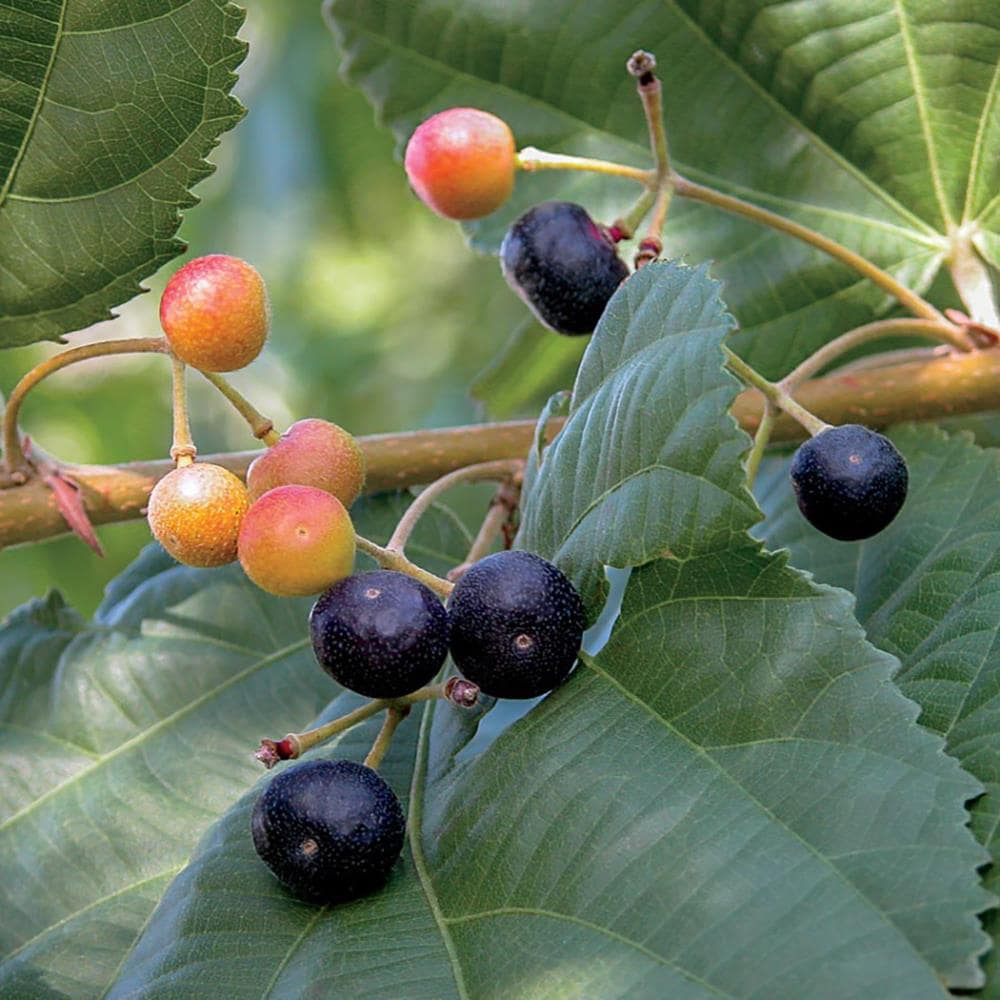The image displays a vibrant outdoor scene with a close-up of a plant. Dominating the foreground are detailed green leaves with sawtooth edges, attached to a central brown branch that diagonally bisects the image from left to right. Sprigs stemming from this branch are adorned with variously colored berries. On the upper left, clusters of light red and orange-yellow berries are prominently visible, suggesting a ripening stage. In contrast, positioned more centrally and toward the lower right, are dark purple and deep red berries, indicative of full ripeness. The background is a soft blur of additional leaves and sunlight, suggesting a sunny day and creating an ambient, natural atmosphere. Dew or rain droplets on the leaves add a fresh, just-rained look to the scene. Overall, the image captures the essence of a natural, outdoor setting with rich colors and textures.